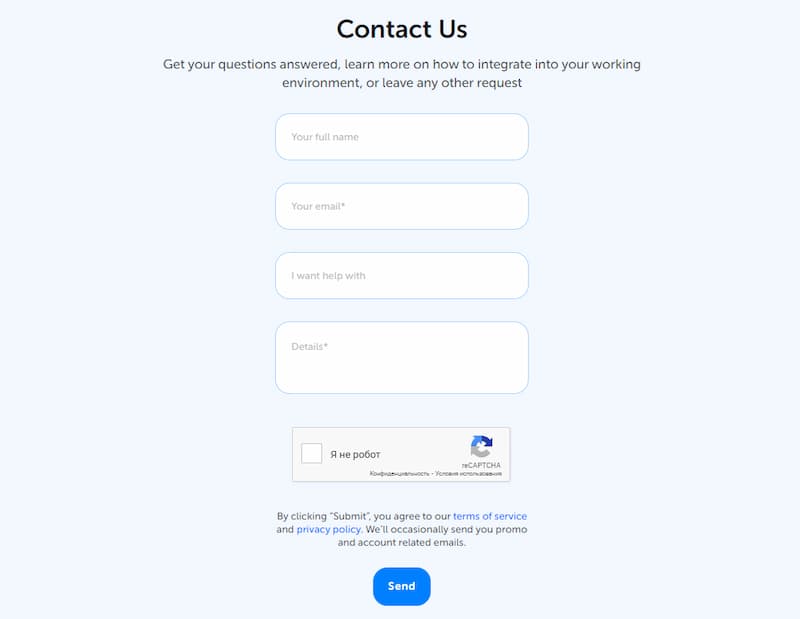The screenshot depicts a structured, light blue contact form designed for user inquiries. The form is square-shaped with a clean, minimalistic aesthetic.

At the top of the form, bold, black, uppercase text clearly instructs "CONTACT US". Directly beneath, slightly smaller text invites users to "Get your questions answered. Learn more on how to integrate into your working environment, or leave any other requests."

Centrally aligned within the blue background, there are four white input fields stacked vertically. These fields are housed in rounded rectangular boxes, each allowing users to fill in specific information:
1. "Your full name" 
2. "Your email"
3. "I want help with"
4. "Details"

Below the input fields is a standard CAPTCHA verification box which includes a grey rectangle and a recognizable CAPTCHA symbol with an arrow making a "C" in blue and gray, signifying the need to complete the CAPTCHA challenge.

At the very bottom of the form, there is a statement in fine print: "By clicking submit, you agree to our terms of service and privacy policy. We'll occasionally send you promo and account-related emails."

Centred at the bottom of the form is a rectangular blue "Send" button, featuring the white text "Send".

Overall, the form is clearly designed to facilitate user engagement through a straightforward and intuitive interface.